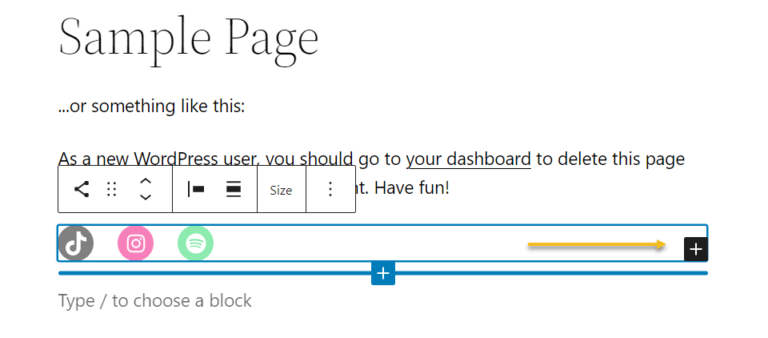Here's a cleaned-up and detailed caption for the described image:

---

The image features a sample page screenshot from a WordPress site. In the top left corner, there is text that reads "Sample Page" with both "S" in "Sample" and "P" in "Page" capitalized. The text is written in a thin font. Directly below, in a slightly smaller and darker black font with increased thickness, it says "...or something like this:". This is followed by the statement "As a new WordPress user, you should go to your dashboard to delete this page." The phrase "your dashboard" is underlined for emphasis.

Further down, the image includes what appears to be a pop-up menu containing several icons. These icons include:
1. A share icon
2. A size icon
3. A justification icon

Below these icons, there are symbols for various social media platforms, specifically:
1. TikTok
2. Instagram
3. Spotify

Lastly, there is an arrow pointing to the right, likely indicating more options or additional content.